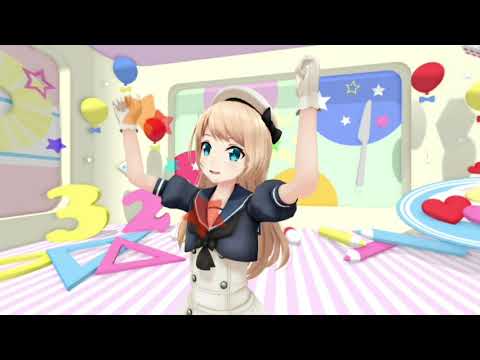The image depicts a female anime character standing front and center, with her hands raised in the air, appearing either surprised or in a celebratory pose. She has large blue eyes and long, light brown hair with a hint of blonde. She is dressed in a blue blouse, adorned with white gloves, and a white dress featuring big buttons. Atop her head is a white cap accented with a black ribbon. The setting is a whimsically decorated room with white and pink striped flooring and beige-ish, white-ish walls. Scattered throughout the room are various colorful, cartoonish objects including numbers (a yellow '3' and a pink '2'), triangles, protractors, and colored pencils in light blue, pink, and yellow. Additional elements include cartoonish forks, knives, stars, a planet, and balloons, creating a lively, kid-friendly atmosphere.